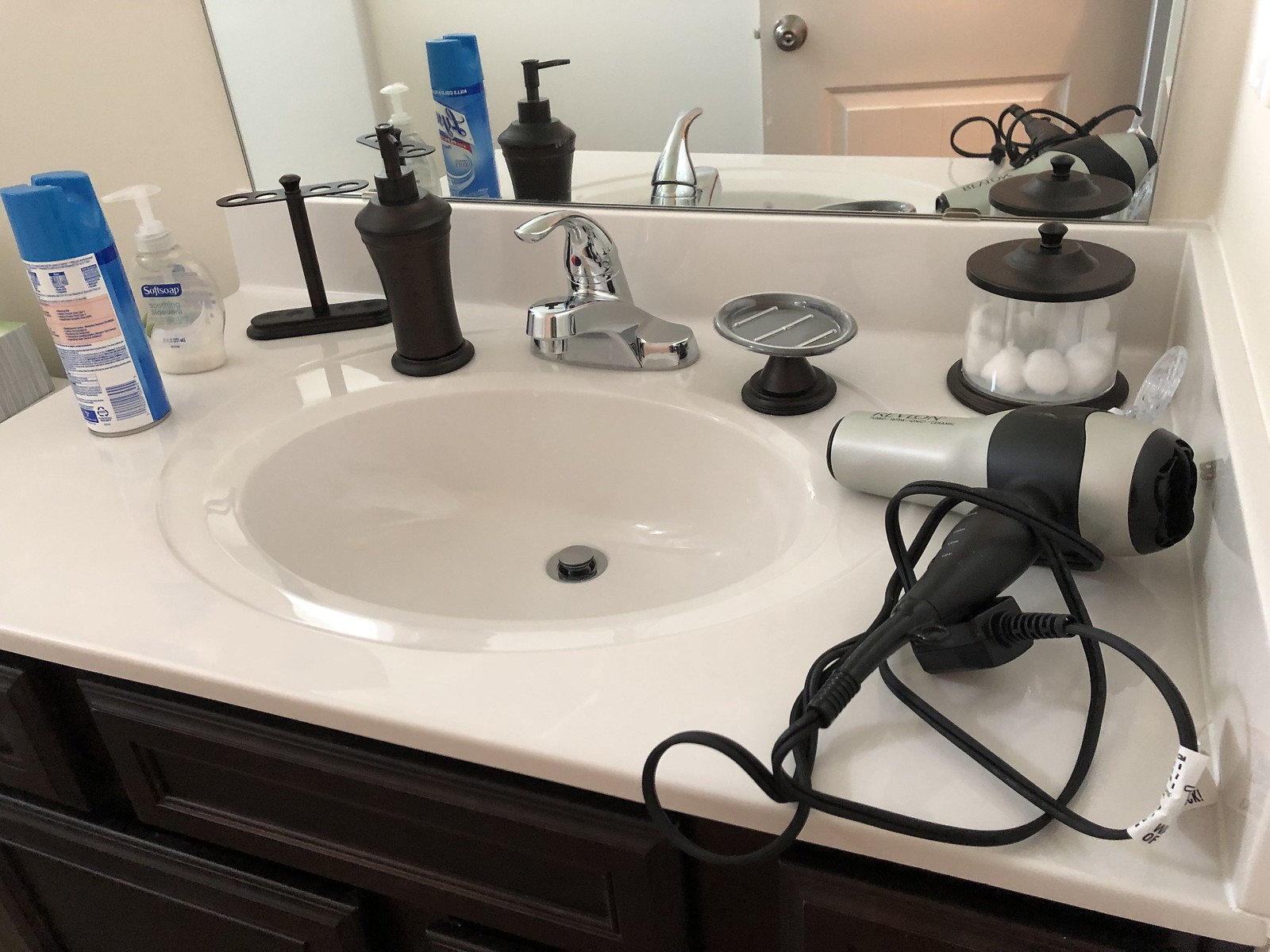In this image, we are viewing a modern bathroom setting with a particular focus on the sink area from a front perspective. The sink is mounted on a black base featuring several individual black drawers, prominently displaying one rectangular drawer at the top center. Above this base sits a white marble sink. 

On the right-hand side of the sink, there is a black hairdryer with a black cord wrapped around it. The hairdryer has a black end, followed by a light gray section, another black segment, and a gray front part. Behind the hairdryer, a black container with a transparent cylinder in the middle, filled with white balls that appear to be cotton, can be seen.

To the left side of the sink, on a black platform, there is a small dish. Adjacent to this is the silver chrome faucet. Further to the left stands a black hand soap dispenser in a vertical position, and next to it is a black stand shaped like an uppercase "I." 

Additionally, a bottle containing white hand soap is positioned to the left of the stand, and next to it is a blue bottle that resembles a Lysol bottle, with a visible white label on the back.